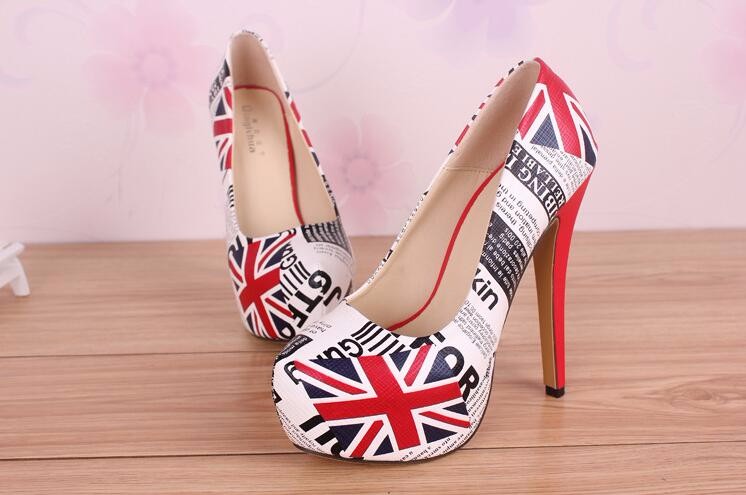The image is a color photograph in landscape orientation showcasing a pair of high-heeled women's shoes positioned on a light brown wooden floor. The shoes are elaborately decorated with a British Union Jack design in red, blue, and white on the front upper part of each toe, accompanied by additional white and black writing along the shoe's surface. The heels are solid red, while the interior lining of the shoes is beige with a prominent red strip where the liner rests against the bottom. One shoe faces the viewer directly, and the other is angled slightly towards the left. The background features a white wall adorned with pink floral wallpaper that has blue accents around the flowers. The image combines elements of photographic realism and product photography, with a slightly off-center and slightly crooked composition, potentially designed for advertisement purposes or personal display.